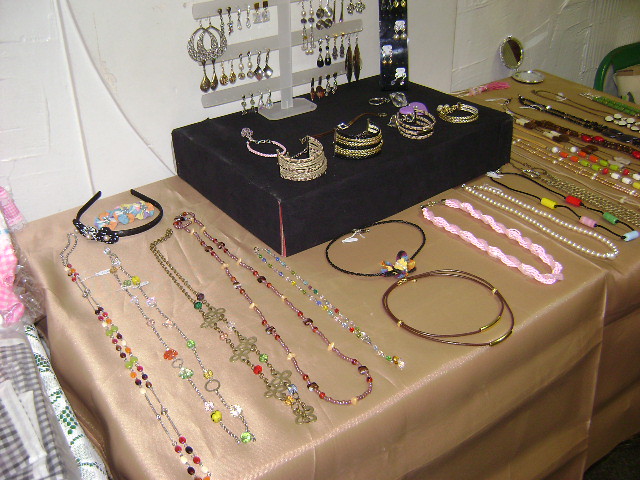This square image captures a detailed setup of a craft fair table laden with an array of handcrafted jewelry. The table, covered with a light brown plastic tablecloth, is adorned with a variety of beaded necklaces, some resembling rosaries, along with pearl and rope-style pieces. In the center back of the table stands a black rectangular box displaying ornate gold bracelets. Atop this box, a white jewelry hanger akin to a tree structure showcases numerous dangly earrings. To the left of this central stand, there's a black headband embellished with sequins. The background features a white wall and, towards the far left, a glimpse of patterned fabric, suggesting the scene is part of a peddler’s or flea market. This meticulously arranged display vividly showcases the diversity and craftsmanship of the jewelry items on sale.